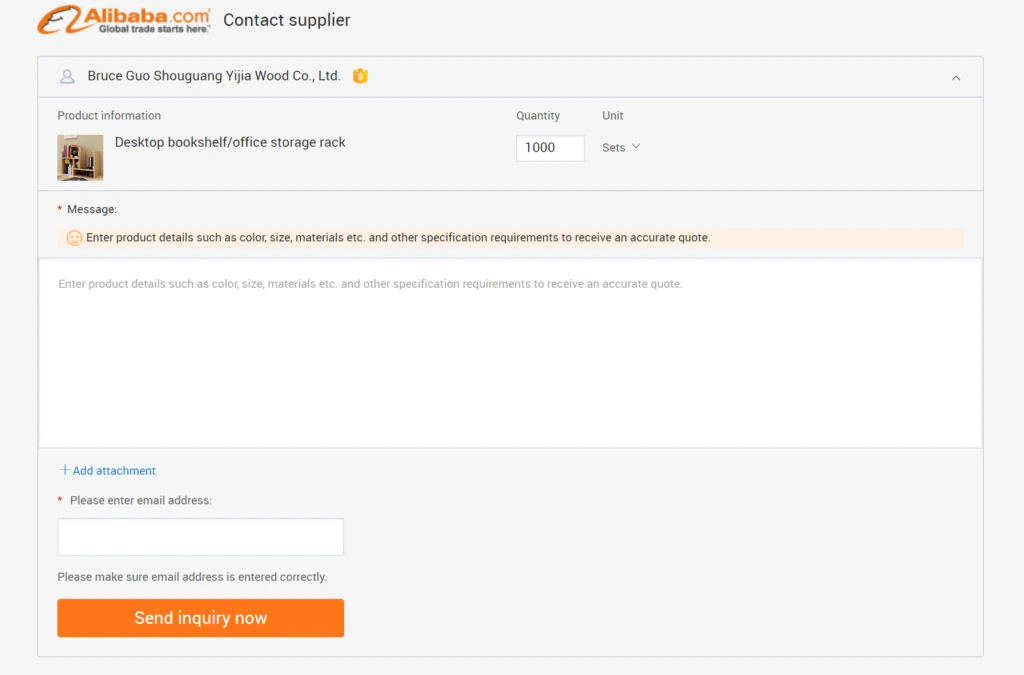This image displays the "Contact Supplier" page on Alibaba.com, showcasing the website's interface and user interaction elements. At the top left, you see the Alibaba.com logo, characterized by its iconic design of an 'A' with a smiley face inside, accompanied by the tagline "Global trade starts here" in orange and black colors.

Central to the image is a prominently displayed, thinly outlined contact form with a gray border. The header of this form features a small human icon alongside the name "Bruce Guo" from "Xiu Guang Yang, Jia Wood Co., Ltd.," highlighted by an orange badge. Below this, under the section "Product Information," there is a photograph of a bookshelf labeled "Desktop Bookshelf/Orange Office Storage Rack" with a listed quantity of 1,000 unit sets.

The message field prompts users to enter specific product details such as color, size, material, and other specifications to receive an accurate quote. Further down, the same prompt text is repeated in light gray within an empty input field.

To the right of this field, there is a blue text with a plus arrow labeled "Add Attachment," allowing users to include additional files. An orange star indicates the necessity of entering an email address, reminding users with a note to ensure the accuracy of their email input within the blank entry field provided below.

Finally, the page features a large orange "Send Inquiry Now" button with white text, mirroring the size of the email entry field and prompting users to submit their inquiry. All sections on the page are clearly separated by thin gray lines, ensuring an organized and easy-to-navigate interface.